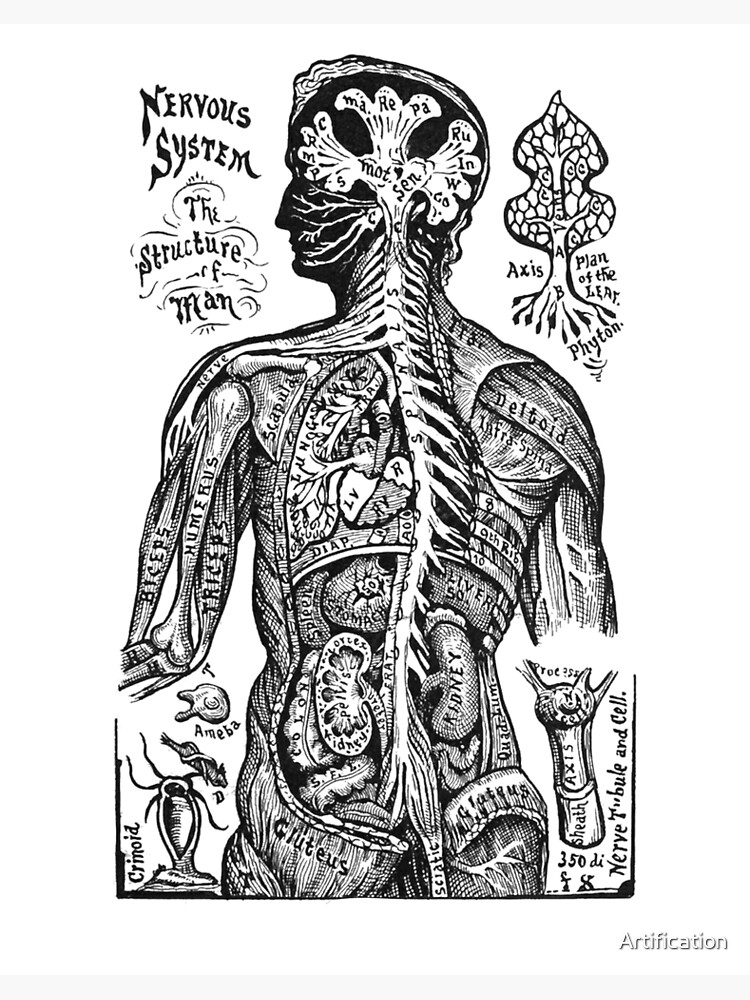This black and white diagram illustrates the human nervous system, titled "The Structure of Man" in the upper left corner. It depicts a human figure from the backside, highlighting various organs, muscles, and bones with intricate labels. The spine is prominently outlined in white, and the brain resembles a piece of cauliflower, annotated with a series of letters. Key anatomical features such as the kidneys, liver, spleen, heart, and gluteus muscles are clearly labeled. Additionally, there are detailed annotations of the bones, including the humerus and biceps. In the upper right corner, there is a section labeled "Axis Plan of the Plant Leaf, Phyton," which includes a drawing of a leaf. The bottom left features labels like amoeba, creating a complex interplay between different biological elements. The artwork provides an educational look at the internal structure of a human, blending scientific accuracy with detailed artistic representation.